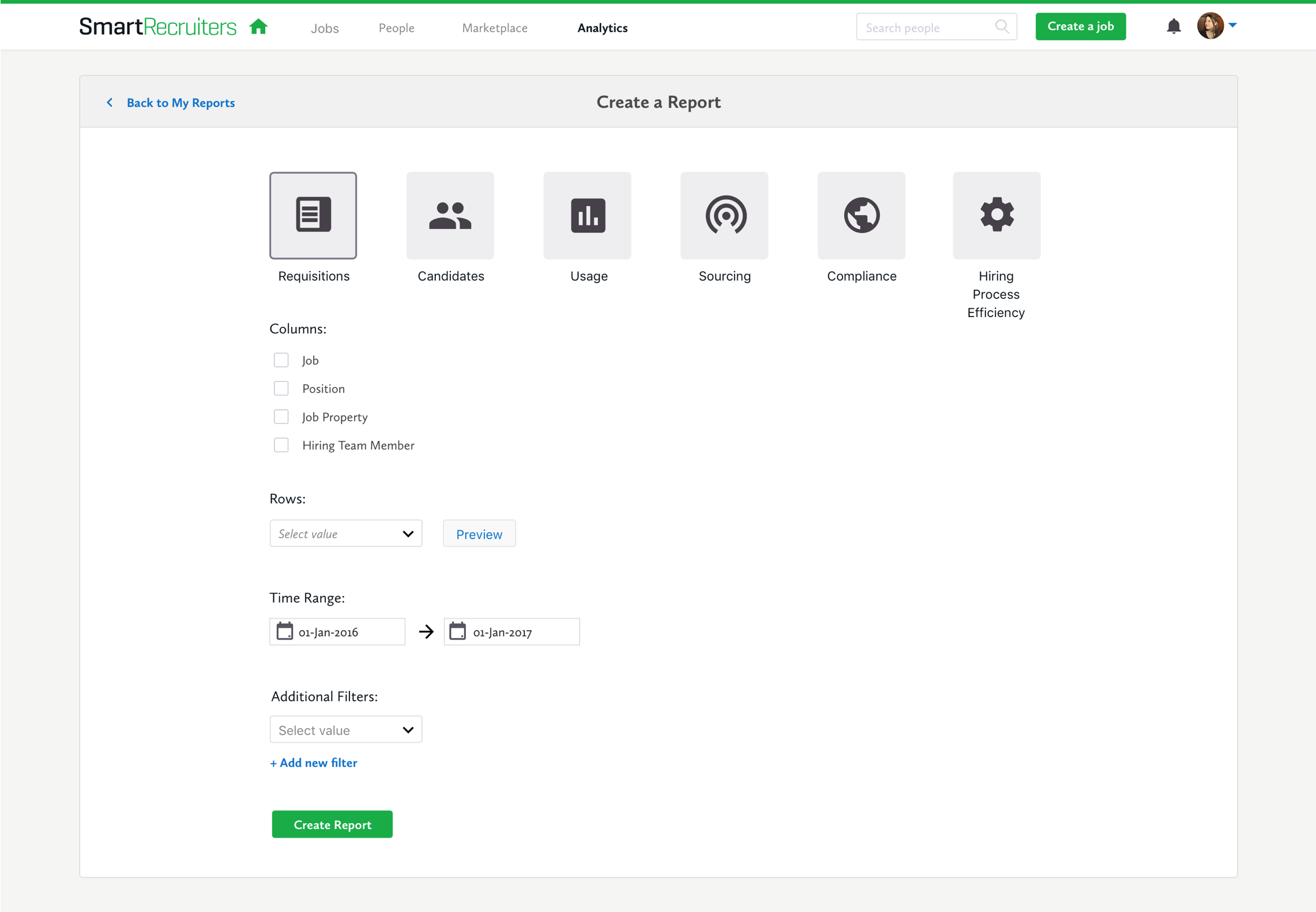**Caption:**

The image features a sophisticated user interface of a recruitment and analytics platform. 

At the top, there's a green border followed by a white background with the branding details. To the left, the word "Smart" is in black, alongside "Recruiters" in green—stylized to resemble a greenhouse. Adjacent to this, in gray, are options: "Jobs," "People," "Marketplace," and "Analytics." 

Below, there is a search bar with a gray outline and a magnifying glass icon inside it. The placeholder text reads, "Search people." Next to the search bar, a green button with white text says "Create a Job." A black bell icon, likely for notifications, is positioned nearby. 

Avatar elements indicating user profiles are present: a female with brown hair facing left, accompanied by a blue triangle. 

The background shifts to gray further down. A significant rectanglular section has a gray and blue top bar. On the left, "Back to Reports" is labeled, and in the center, the text "Create a Report" is in black. 

Within this section are multiple labeled gray boxes: "Requisitions," "Candidates," "Usage," "Sources," "Compliance," and "Hiring Process Efficiency." Various columns feature headers such as "Job Position," "Job Property," "Hiring Team Member Roles," and "Select Value." Next to this, there's a gray rectangle with the word "Preview" in blue. 

The time range section is in black text with selected dates "01-January, 2016" and "01-January, 2017," indicated by a black arrow. An additional filter box in gray prompts users to "Select Value," with a blue link below it to "+ Add New Filter."